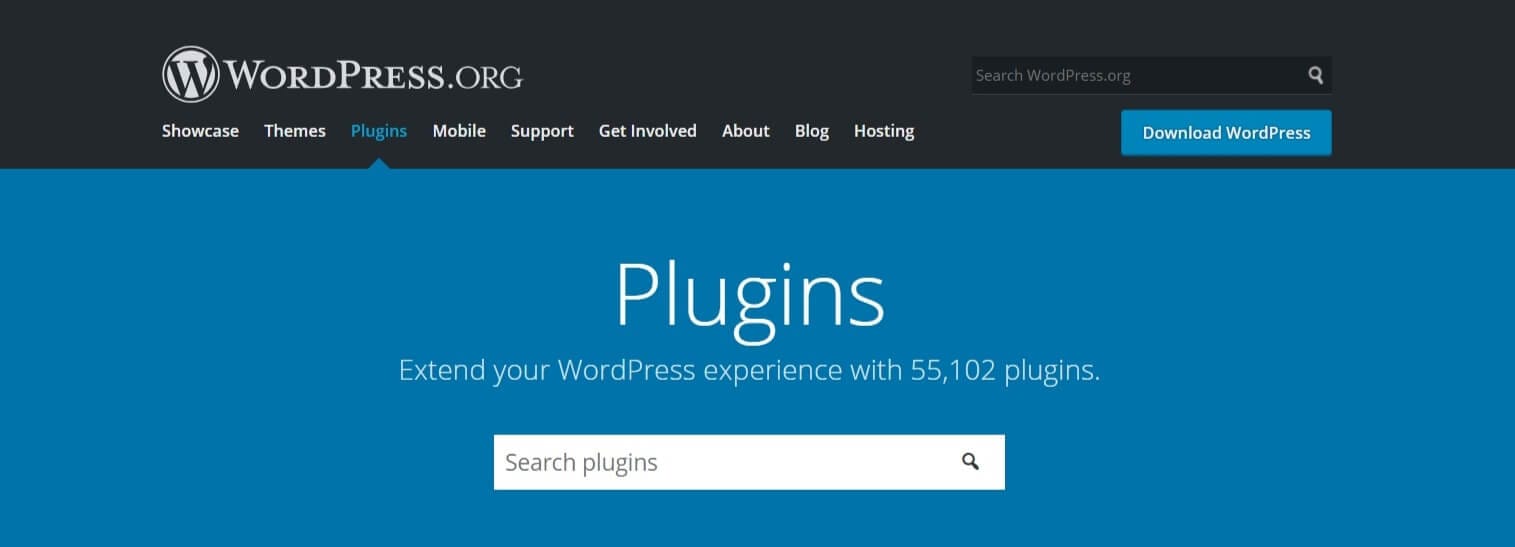This is a screenshot of the plugins section on wordpress.org. At the top, you can see the wordpress.org logo featuring a monochrome "W" encased in a circle, which blends seamlessly with the dark gray navigation bar. On the right side of this bar, there is a search field labeled "Search wordpress.org" and beneath it, a prominent blue button with the text "Download WordPress."

To the left, there’s a vertical navigation menu with several options in white text: Showcase, Themes, Plugins (highlighted in blue), Mobile, Support, Get Involved, About, Blog, and Hosting. The highlighted Plugins option is emphasized by a blue field stretching the full width of the screenshot and a blue triangle at the top, pointing directly at the Plugins label.

In this blue section, large white text reads "Plugins", below which, in smaller white text, it states: "Extend your WordPress experience with 55,102 plugins." Directly beneath this is a search bar for finding specific plugins, featuring a white input field with a subtle gray magnifying glass icon on the right side.

The screenshot captures just this upper portion of the plugins page, providing a concise overview with no further content appearing below the search bar.